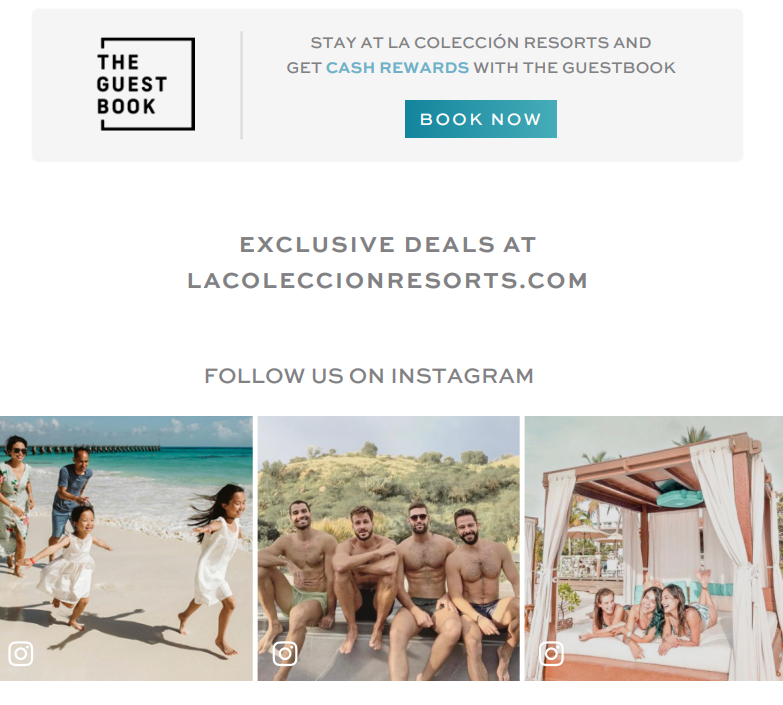This advertisement for La Coliseum Resorts prominently features a promotion for "The Guest Book" in the top left corner, enclosed within a black box icon. To the right, bold text invites viewers to "Stay at La Coliseum Resorts and get cash rewards with The Guest Book." Below this, a teal call-to-action button with white text urges users to "Book Now." The caption highlights "Exclusive deals at La Coliseum Resorts" and encourages following their Instagram account for updates.

The advertisement includes three Instagram-marked photos:
1. The first image captures an Asian family enjoying a beach day. The family consists of a husband, wife, and two young daughters all running along the shore. The daughters are dressed in white dresses, the man wears a blue shirt paired with blue shorts, and the woman is in a light blue or green floral dress.
2. The middle photo features four men, all wearing swimsuits without shirts, smiling warmly at the camera. The man third from the left sports sunglasses, and all four men have beards.
3. The third image shows three younger women lounging in an outdoor cabana or bed, laughing together. The cabana is shaded with an awning and curtains that can be drawn for privacy.

This vibrant and inviting advertisement aims to showcase the enjoyable and diverse experiences available at La Coliseum Resorts.